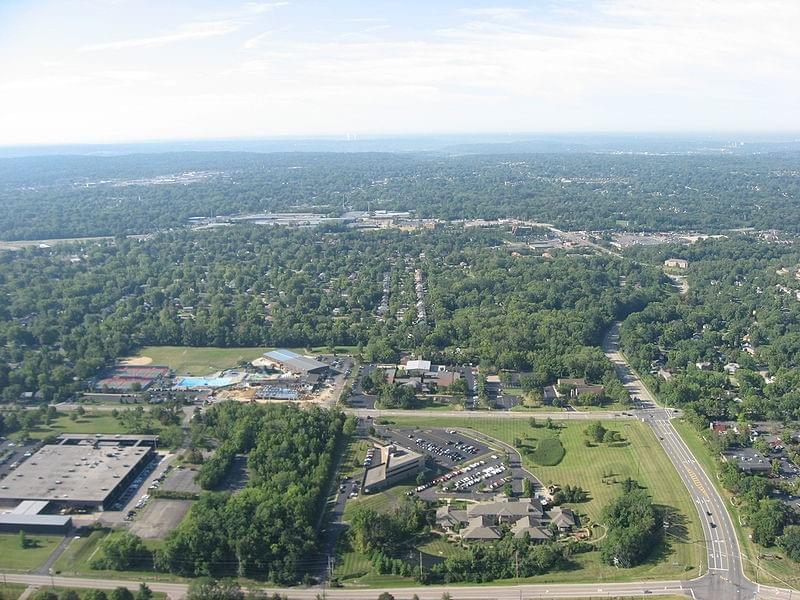This detailed aerial image captures a scenic view of a city set against a backdrop of natural beauty. The photograph, likely taken from a drone or helicopter, showcases a sprawling urban landscape surrounded by dense, verdant forests and lush greenery. The foreground features a bustling campus-like area with large office and industrial buildings, their adjacent parking lots filled with numerous cars. Roads and highways weave through the city and forest, with visible yellow and white road lines and moving vehicles.

In the distance, the skyline presents a contrast of natural and urban elements: a light blue sky adorned with delicate, whispery clouds, and a mountainous region blanketed in blues and greens. The upper portions of the image hint at dark blue waters, while further back, scattered houses and buildings become visible among the dense forestry. Amenities like a pool and tennis courts suggest a recreational center within the scene. The overall clarity of the day, with some wispy clouds, ensures a bright and vivid capture of this harmonious blend of city and nature.